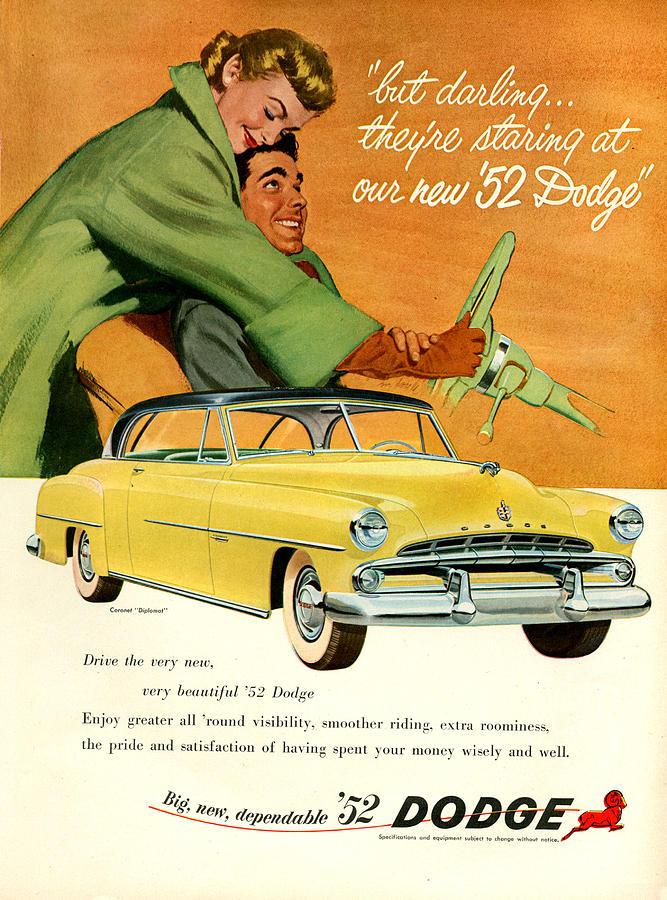The advertisement, likely from the 1950s, showcases the new 1952 Dodge car in a full-page format. The upper half of the ad features an illustration with an orange background depicting a joyous couple in the car. The man with dark hair and a big smile is in the driver's seat, looking lovingly up at the woman behind him. She is a beautiful blonde with red lips, dressed in a big green coat, and embraces him warmly. Above them, in white cursive text, the ad reads, "But darling, they're staring at our new 52 Dodge."

Prominently placed in the middle of the advertisement is a large yellow Dodge car with a black top, epitomizing classic 1950s design. Below the car, a beige background with black text invites potential buyers: "Drive the very new, very beautiful 52 Dodge. Enjoy greater all-round visibility, smoother riding, extra roominess, the pride and satisfaction of having spent your money wisely and well." The ad concludes with bold text curving upward, stating, "Big new dependable 52 Dodge," next to a small red ram logo, which symbolizes the Dodge brand.